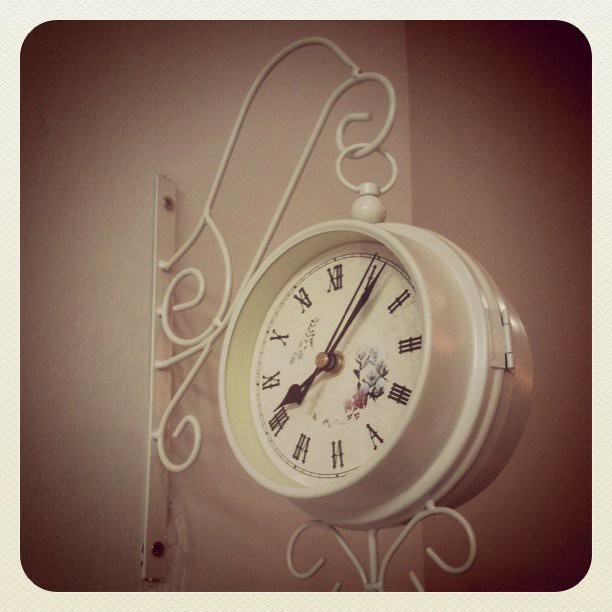A beautifully crafted analog clock adorns the interior wall, giving an exquisite touch to the decor. The clock is suspended from a slender, wrought iron panel securely fastened to the wall with visible screws. Elegantly painted iron scrollwork emerges from the panel, gracefully framing the clock. The clock, fashioned from a white-toned metal, features a pristine white face adorned with Roman numerals. Delicate floral and leaf motifs add a charming, vintage appeal to its design. More intricate white iron scrollwork delicately dangles from the base of the clock, enhancing its ornate and timeless aesthetic.